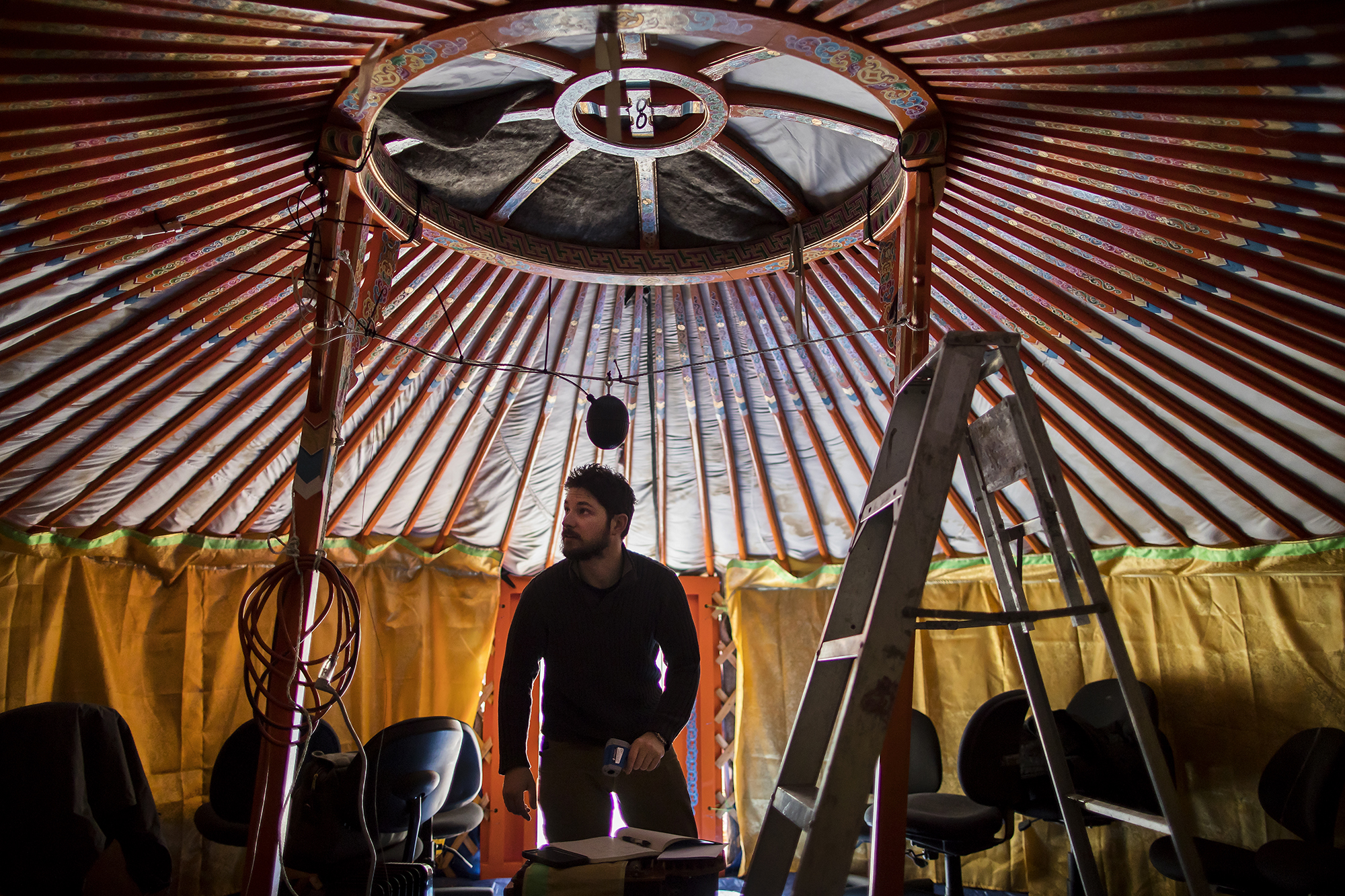In the center of this image, a man with a beard and short black hair stands inside a circular yurt. The roof of the yurt features wooden beams arranged in slats that converge at a central circular hub, resembling a hubcap. This central circle has a smaller circle within it and radiating spokes. The man, dressed in a black long-sleeved shirt and dark pants, is holding a blue laser stud finder and is looking to his left. The lower portion of the yurt's walls is draped with yellow curtains bordered by a light green trim at the top. A light brown, four-rung stepladder is positioned to the right of the man, and in the background, several office chairs with black cushions, an open book, and extension cables are visible. These additional items suggest a combination of living and work space within the tent-like structure.